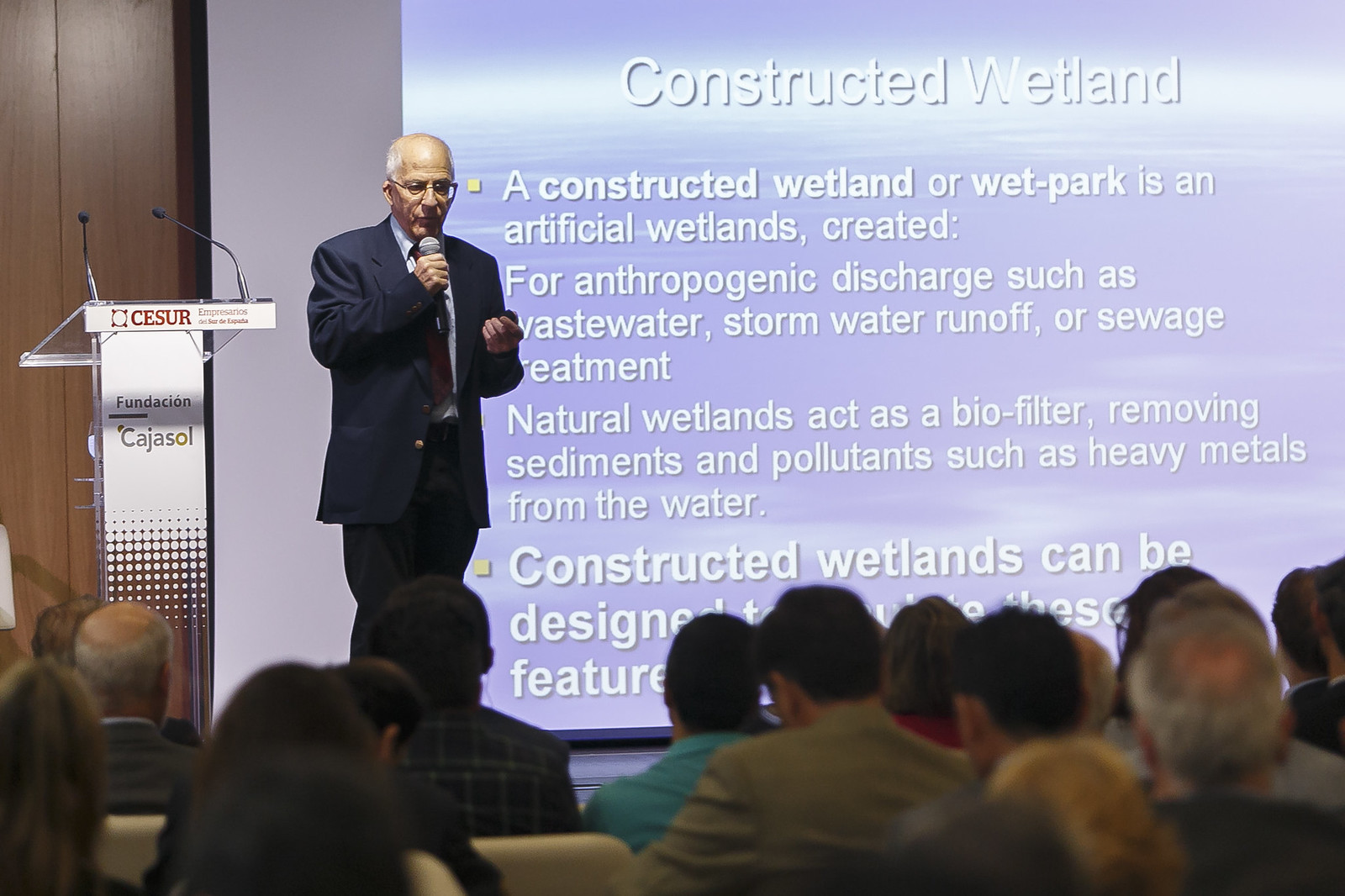An older white man, bald except for the edges of his head, stands on a stage giving a presentation. Dressed in a loose-fitting suit and tie, he holds a wireless microphone in his right hand. He is wearing glasses and is positioned near a white podium. Behind him is a large projector screen displaying a PowerPoint slide with a blue and white background. The title of the slide, "Constructed Wetland," appears prominently at the top. The visible text on the slide reads, "A constructed wetland or wet park is an artificial wetland created for anthropogenic discharge such as wastewater, stormwater runoff, or sewage treatment. Natural wetlands act as a biofilter, removing sediments and pollutants such as heavy metals from the water." The bottom of the slide text is cut off, but visible words include "constructed wetlands can be designed." The focus of the photograph is on the presenter, with several rows of older adults visible and slightly out of focus at the bottom edge of the image, attentively watching the presentation.